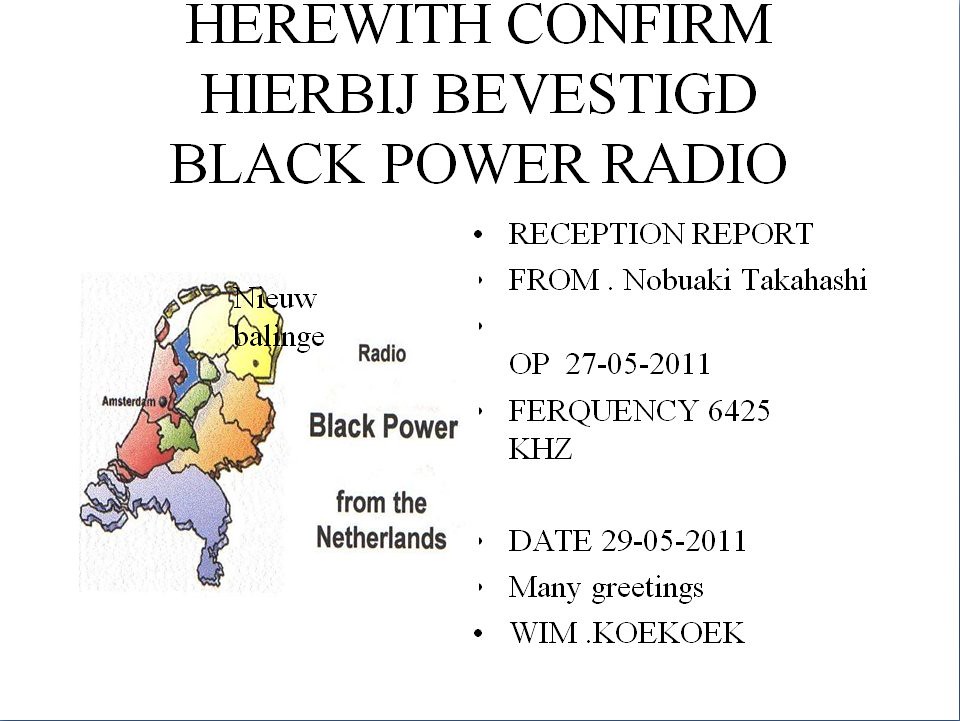The image is a detailed reception report for "Black Power Radio" from the Netherlands, set against a white background. At the top of the report, in large, bold, black capital letters, it reads: "HEREWITH CONFIRM," followed by Dutch text: "HIERBIJ BEVESTIGD," and "BLACK POWER RADIO." The report further details the reception report from Nobuaki Takahashi with specifics: OP27-05-2011, Frequency 6425 kHz, and the date 29-05-2011. It concludes with the sender's name, "Many Greetings, Wim Koekoek." In the center of the graphic, there is a mention of "Radio Black Power from the Netherlands." Additionally, the report features a colorful, detailed digital graphic of a map of the Netherlands with marked locations, including Amsterdam and Nieuwe Balinge, positioned mostly at the northernmost part of the country. The graphic is bordered by a thin black line on the right and bottom sides.